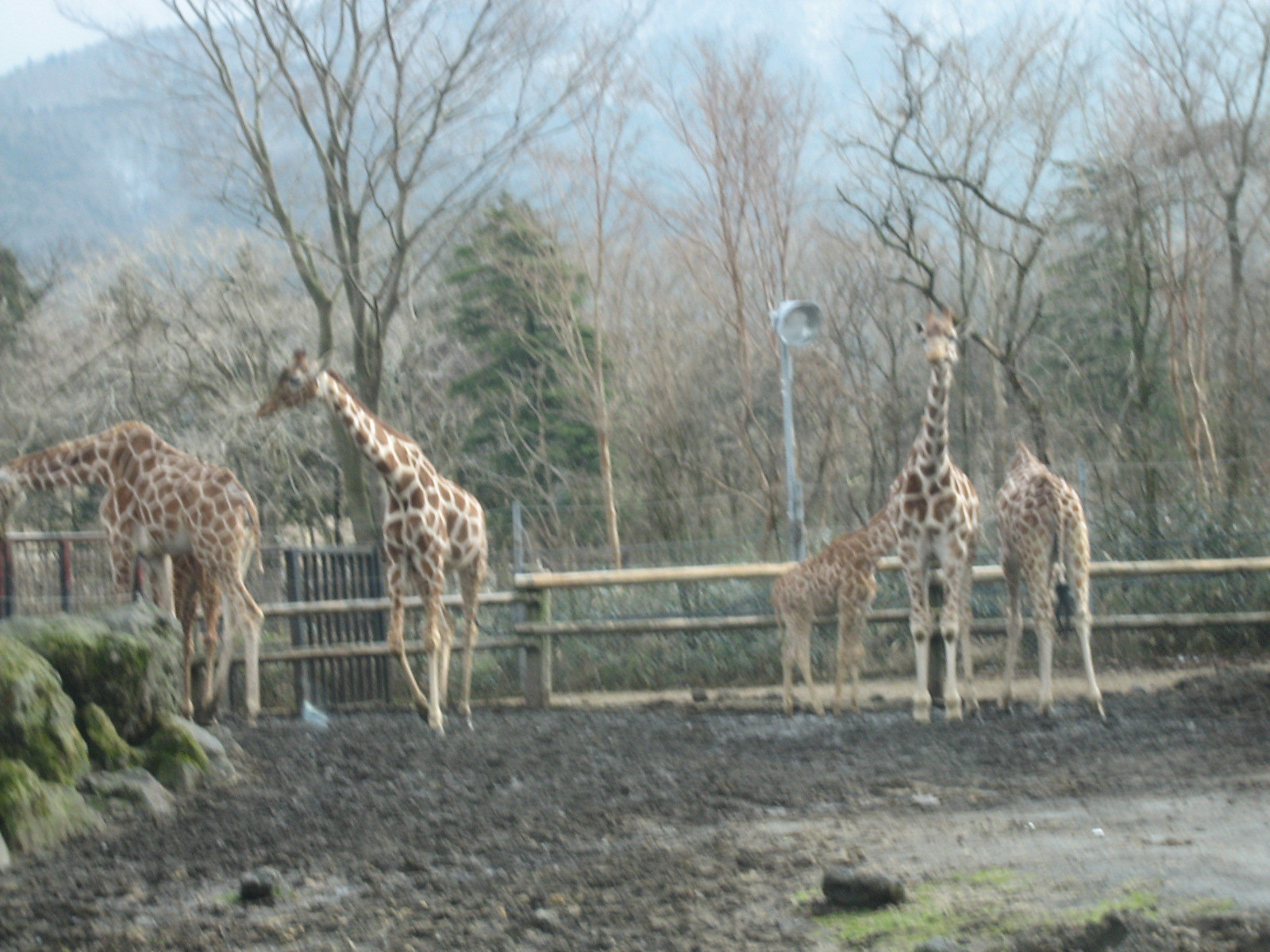This slightly blurry photograph captures a group of five giraffes in a zoo or country park. The giraffes are in a large, muddy enclosure with a wooden fence that reaches about halfway up their bodies. On the left side of the image, two giraffes are clustered together; the far-left one is leaning over the fence, while the one next to it is walking towards the viewer but looking to the left. A small rock outcropping and mossy rocks can also be seen on this side. In the center-right of the image, there are three more giraffes. The middle giraffe of this group is facing directly at the camera, with a giraffe to its right facing away and another smaller giraffe partially obscured behind it. Surrounding the enclosure is a backdrop of trees, mostly barren except for one possible fir tree, creating a wild yet somewhat stark atmosphere. In the distant background, a fog-covered mountain adds to the cold and muted feel of the scene. The photograph does not have any text or identifying markers to indicate its location.